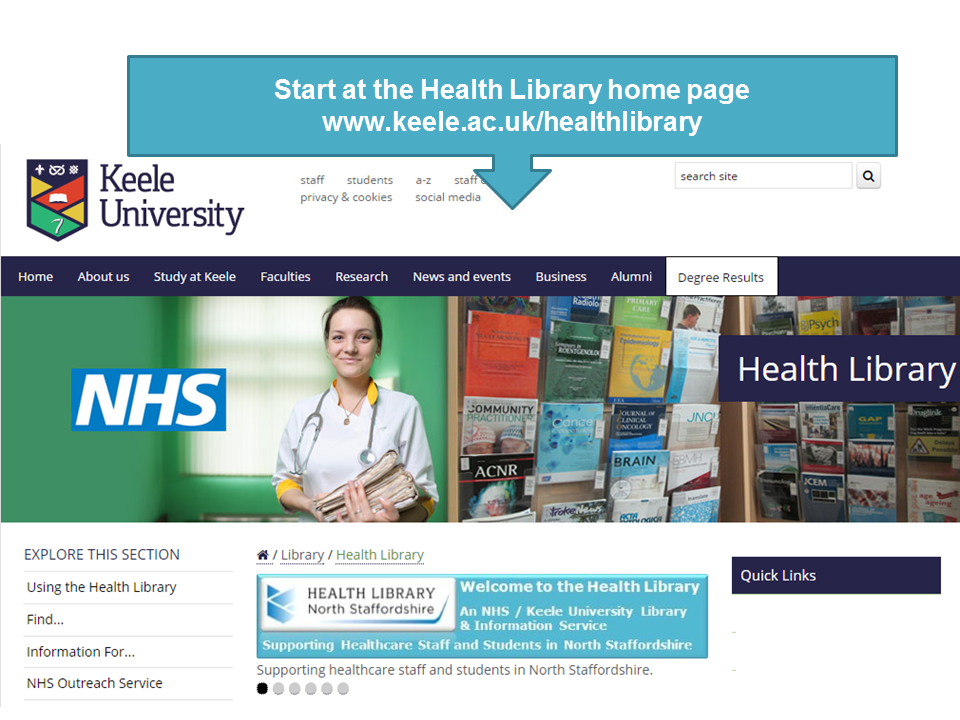The webpage for Keele University Health Library features a structured and detailed layout designed for easy navigation. At the top, a directive invites users to "Start at the Health Library Homepage" followed by its URL: www.keele.ac.uk/healthlibrary. Beneath this, a horizontal menu bar includes the Keele University logo and an array of options: "Staff," "Students," "Privacy and Cookies," "A-Z," "Staff" again, "Social Media," and a convenient search box on the far right.

A secondary navigation strip below offers links to primary areas of the site: "Home," "About Us," "Study at Keele," "Faculties," "Research," "News and Events," "Business," "Alumni," and "Degree Results." Directly below this navigation bar are two images; the left one depicts a young white woman in a nursing uniform, and the right image consists of reading materials with the words "Health Library" superimposed.

Further down the page, the left sidebar guides users with the text: "Explore this section using Health Library, find information for an NHS outreach service." In the center, a welcoming message reads "Health Library, Health Library North Staffordshire, Welcome to the Health Library at NHS Keele University Library and Information Service, supporting healthcare staff and students in North Staffordshire." This message is reiterated below for emphasis.

On the far right of the page, a dark blue box labeled "Quick Links" in white text offers easy access to essential resources. The page's design ensures that users can easily find and navigate to the information they need, whether they're healthcare staff, students, or visitors seeking specific services or resources provided by the Keele University Health Library.